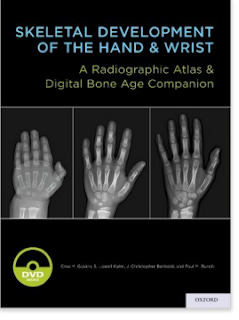The image displays the cover of a DVD case, primarily black, featuring three different hand x-rays. At the top, in uppercase light blue text, it reads "Skeletal Development of the Hand and Wrist." Directly below that, in smaller light yellow text, it states "A Radiographic Atlas and Digital Bone Age Companion." The central section showcases the three x-rays: the left one showing a hand with fingers close together, the middle one with a slightly more open, fully extended hand, and the right displaying a larger, fully extended hand with fingers spread out. Beneath these images, a neon green DVD icon appears, accompanied by some unreadable text. In the bottom right corner, a white rectangle contains the word "Oxford" in black.